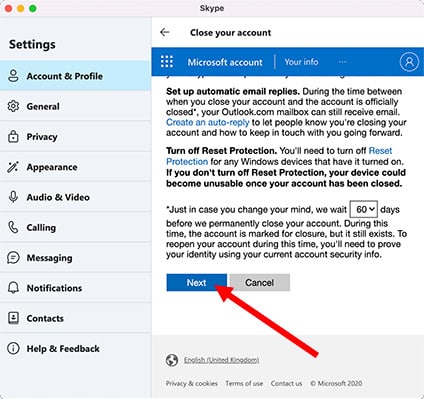The image depicts a screenshot of a Skype settings page on a Mac running macOS. The left side of the window displays a vertical menu with various setting categories including 'Account and Profile,' 'General,' 'Privacy,' 'Appearance,' 'Audio and Video,' 'Calling,' 'Messaging,' 'Notifications,' 'Contacts,' and 'Help and Feedback.'

The user has selected 'Account and Profile,' revealing a detailed page titled "Close Your Account." While most of the content is off-screen, the visible section details two important actions: setting up automatic email replies and turning off reset protection for Windows devices.

The first section explains that users can configure automatic email replies during the interim period between initiating account closure and the account being officially closed. This allows users to inform contacts of the impending account closure.

The second section advises users to disable reset protection for any Windows devices linked to the account to prevent them from becoming unusable post-account closure.

Additionally, the page mentions a 60-day grace period, starting from the account closure request, during which the account is marked for closure but not yet permanently deleted. During this period, users can reactivate their account by verifying their identity with current security information.

At the bottom of the page, there are two buttons: 'Next,' in blue, which likely advances the process, and 'Cancel,' which aborts it.